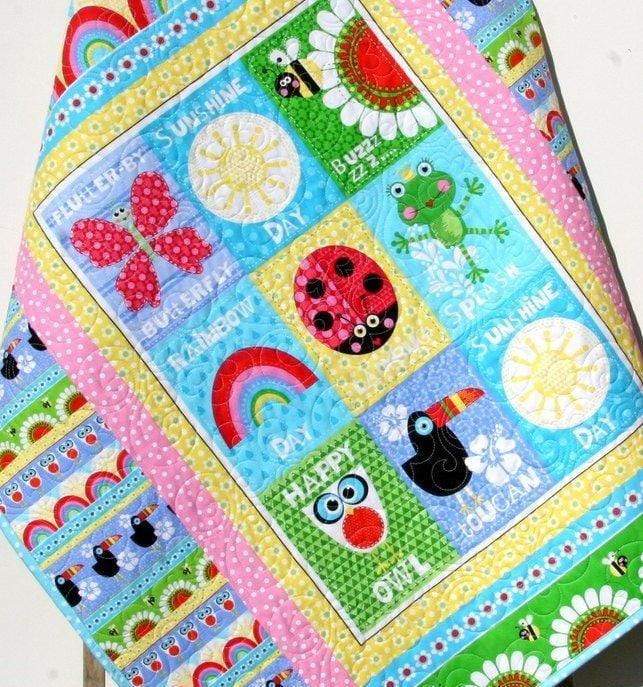This photograph features a colorful baby quilt, likely draped over the back of a chair or hanging on a hook, as the sides curve backward slightly. The quilt's background displays a white surface, possibly the chair itself. Crafted in a patchwork style, the center of the quilt is decorated with various squares, each showcasing vibrant cartoon images and text. Prominently positioned in the middle, a ladybug square labeled "Happy" sits next to a frog captioned "Splash" on the right and a rainbow marked "Rainbow Day" on the left. Below the ladybug, a toucan square and a square with a white owl and blue eyes are visible, the latter labeled "Happy Owl." The bottom right showcases a sun square with the text "Sunshine Day." 

The top row features a butterfly square labeled "Flutter By" on the left, a second sun square with "Sunshine Day" in the center, and a bee with the caption "Buzz Buzz" next to a flower on the right. The quilt is emphasized with multicolored borders, incorporating light pink, yellow, light blue, and dark green hues. Colors used in the quilt include yellow, brown, blue, pink, purple, black, white, orange, and green. Smaller versions of these cartoon images are scattered around the edges, enhancing the quilt's playful and detailed design.